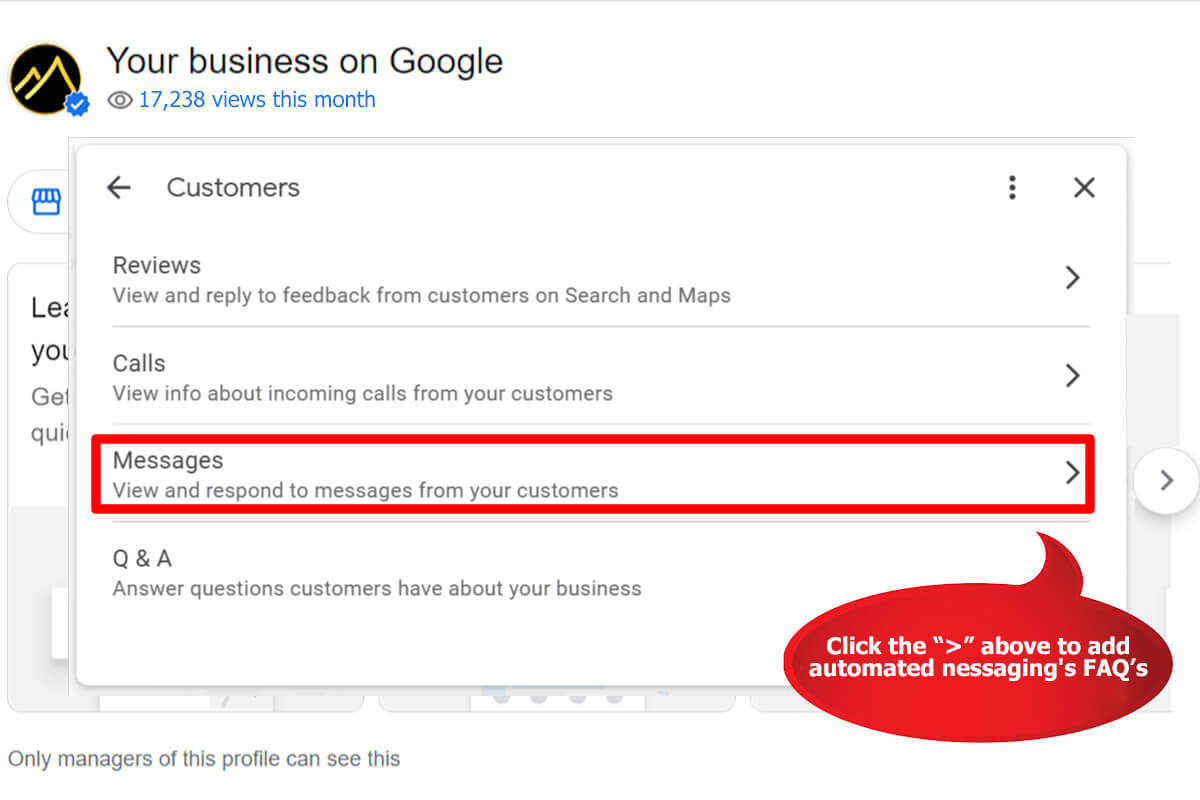This is an image of a web page titled "Your Business on Google," prominently displayed in the upper left-hand corner of the screen. Adjacent to the title is a black circular logo featuring two gold-outlined mountains within the black circle. Below the title, the page highlights the visibility of the business with a statistic, stating that it has received 17,238 views this month.

Following the view count, the customer portal is detailed with various sections. The first section is titled "Reviews," under which it instructs users to "View and Reply to Feedback from Customers on Searches and Maps." Directly beneath this, the "Calls" portion provides information with the directive to "View Info about incoming calls from your customers."

Further down, a section titled "Messages," distinctly circled in red, emphasizes the ability to "View and Respond to Messages from Your Customers." At the bottom of the portal, there's a "Q&A" section designed for business-related inquiries, indicated by a dialog box feature catering to customer interactions on the business website hosted by Google.